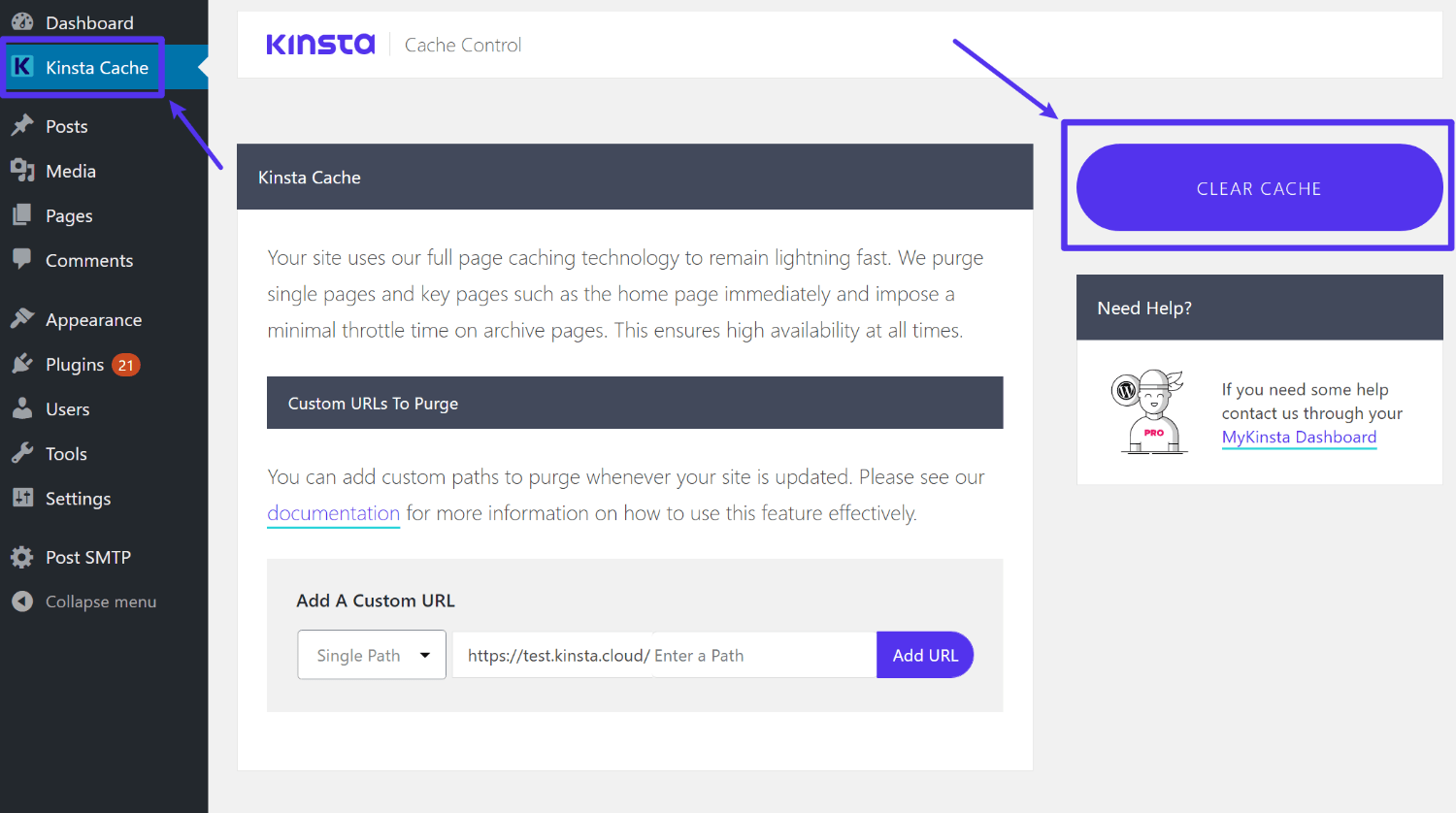On the far left-hand side of the image, there is a vertical black rectangle with the word "Dashboard" written in white text at the top. Below this, a list of menu options can be seen: Kinsta Cache, Posts, Media, Pages, Comments, Appearance, Plugins, Users, Tools, Settings, Posts, SMTP, and Collapse Menu. Each of these options features an icon to its left representing its function.

The Kinsta Cache option stands out with a blue rectangular background, further highlighted by a purple-outlined rectangle around it. This rectangle includes an arrow pointing up toward the bottom right corner. An orange counter next to the Plugins option displays the number "21."

In the main section of the screen is a white rectangle labeled "Kinsta Cache Control." The word "Kinsta" is written in a purple font, positioned near an arrow pointing downwards towards the "Clear Cache" button, which is also purple with a purple border rectangle.

Below the "Kinsta Cache Control" section, there is a segment titled "Kinsta Cache Information" with text in gray and several dark bluish-gray rectangular boxes. Toward the bottom of the image, there is an option to add a custom URL, accompanied by a drop-down arrow and a field labeled "Single Path" with a space for a URL link. Adjacent to this field is a purple button labeled "Add URL."